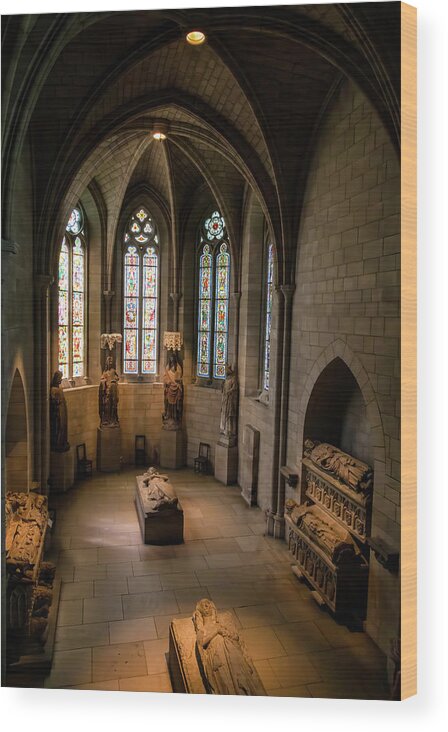This detailed wall art photograph captures the intricate and medieval interior of a Gothic-style church, showcasing the solemn atmosphere of a mausoleum. The church, made of greyish-brown stone, features high, arched ceilings in the Victorian style, giving the room a narrow yet elongated appearance. 

The central focus is on three tall, narrow arched stained glass windows, primarily white or translucent with hints of red, casting a muted light into the space. At the room's center lie two stone sarcophagi, resembling mummy beds, each adorned with statues of deceased figures, suggesting they contain corpses. Additional arched recesses on both the left and right walls also house stone coffins, each topped with statues of the interred.

The room's floor is covered in square or rectangular tiles, and the lighting is further supplemented by small, circular windows near the arched roof. The photograph, rectangular in shape and approximately 5 to 6 inches high and 2 to 3 inches wide, is mounted on a wooden backing, creating a slight shadow effect on the right side. The absence of a border adds to the image's immersive depth, drawing viewers into its meticulously detailed depiction of Gothic funerary architecture.